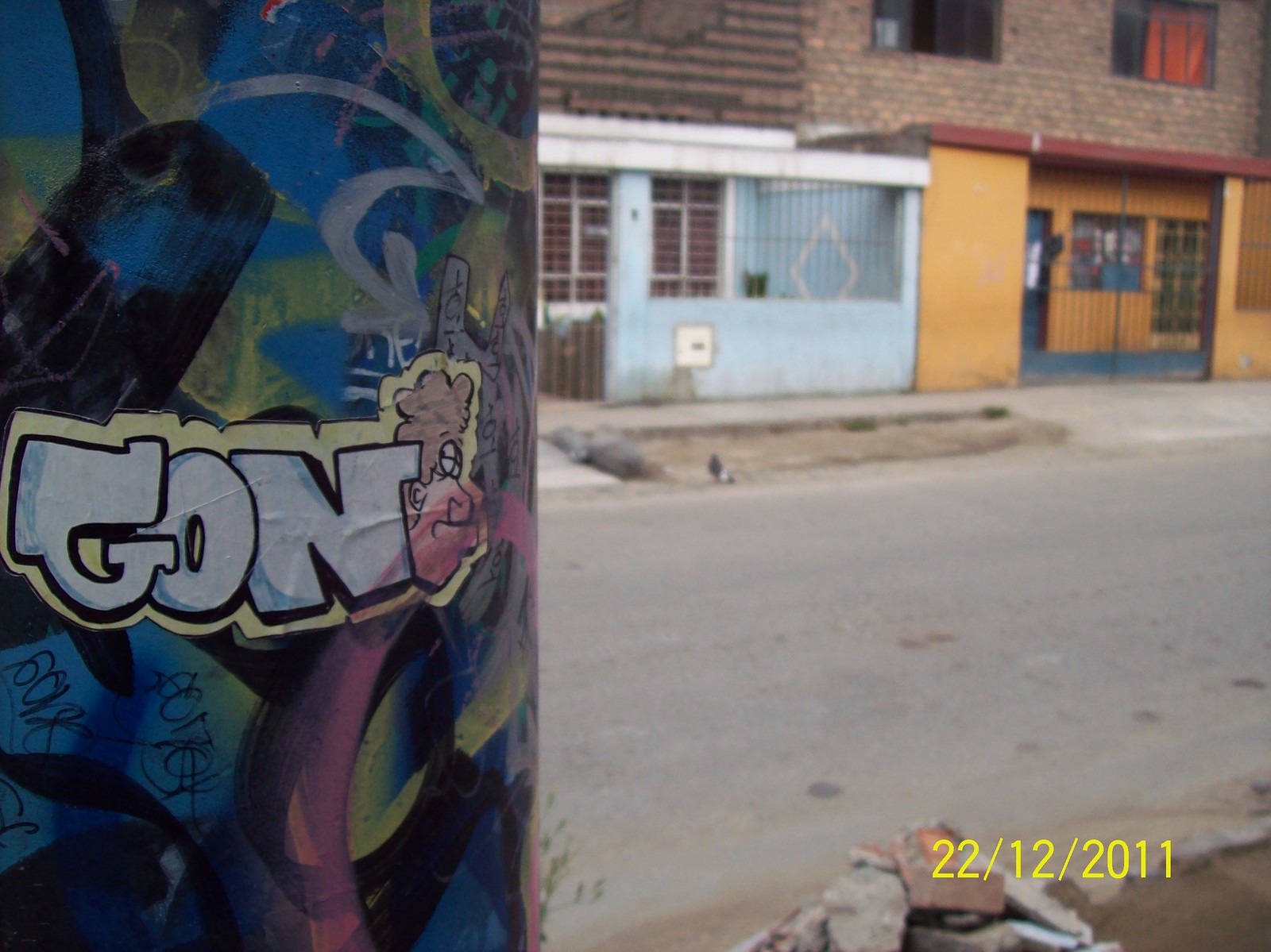This image captures an outdoor scene during the day, centered around a stone or concrete street that runs horizontally across the center. The setting includes detailed structures and objects on both sides of the street. On the left side, there is a vividly painted pole adorned with various colors such as blue, red, yellow, black, and a sticker showing a face and blocky graffiti-like white text reading "G-O-N." 

Moving to the right side of the image, a collection of buildings comes into view. Dominating the scene is a yellow building on the lower level, featuring a blue doorway and a black gate. Above this level sits a brick structure characterized by two large windows. Adjacent to this is a light blue building with a distinct white diamond shape on its wall, further accented by a red structure behind it. A small strip of gray sidewalk lies in front of these buildings, separating them from the street.

The surface of the street shows some spots, possibly from oil drips or dirt. A noticeable pile of dirt is present in the bottom right corner of the image. The only text visible within the scene is a date, "22-12-2011," located in the bottom right corner. The diverse color palette of the image includes shades of blue, green, yellow, tan, brown, black, white, orange, and red, providing a visually rich and detailed view of a typical street scene.